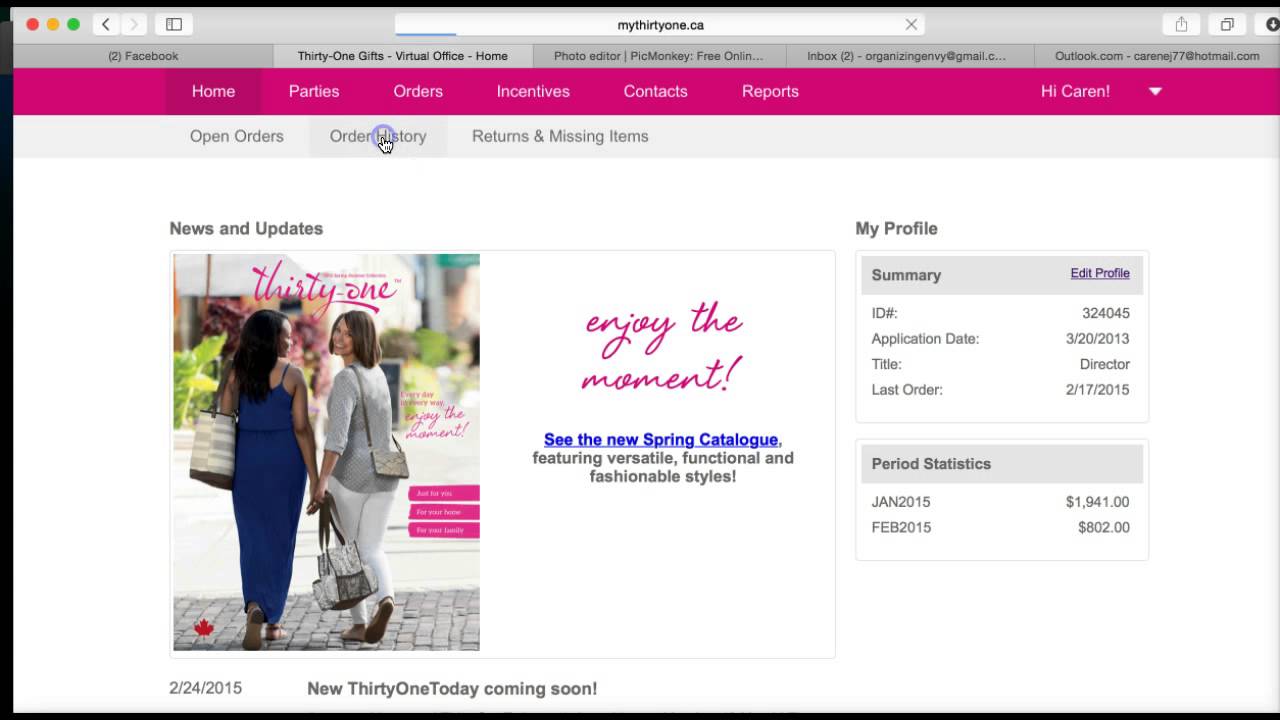This image is a detailed screenshot of a website displayed in the Safari browser. At the top, the familiar Safari user interface is visible, including the red, yellow, and green traffic light buttons on the left, along with the back and forward navigation buttons, history, and bookmark functions. The browser's white address bar prominently displays "my31.ca" in black text, with a grey 'X' on the far right. Multiple tabs are open beneath this bar: Facebook, 31 Gifts - Virtual Office: Home, a Video Editor application, PicMonkey, and two email services (Gmail and Outlook).

The main content of the website starts with a bright pinkish-purple navigation bar, holding options like Home, Parties, Orders, Incentives, Contacts, and Reports, all in white text. The Home button appears highlighted in a darker shade of pink. On the right end of this navigation bar, it greets the user with "Hi Karen!" followed by a white downward arrow for more options.

Below this pink navigation bar, a secondary, light grey menu displays options such as Open Orders, Order History, and Returns and Missing Items, with the cursor currently hovering over "Order History."

The primary section of the website features a white background. On the left, under the heading "News and Updates," there's a rectangular box with a thin grey border. Inside, an image captures two women walking, viewed from behind. One woman, with brunette hair, wears a long blue sundress or jumpsuit with spaghetti straps and carries a large white and grey striped tote bag. The second woman, with shoulder-length brown hair, wears a grey quarter-sleeve button-down shirt paired with white pants, a square grey purse slung over her shoulder, and holds several bags in her hand. She smiles back at the camera. Above the image, "31" is written in cursive pink letters. To the right of the picture, in a white box, the text reads "enjoy the moment" in pinkish-purple font, followed by a blue link that says "see the new spring catalog" and a subtext in black explaining it's featuring versatile, functional, and fashionable styles.

Below this rectangular information box, the date "2/24/2015" along with the phrase "new 31 today coming soon" is displayed.

Adjacent to the news section on the right, an order summary box is present. The top heading states "My Profile," followed by two subdivided rectangular boxes with grey borders. The first box, titled "Summary," has an "Edit Profile" link in purple. Inside, it lists an ID number (324045), application date (3/20/2013), title (Director), and the last order dated (2/17/2015). The second shorter box is titled "Period Statistics," showing financial statistics for two months: January 2015 ($1,941) and February 2015 ($802.00).

The entire image is surrounded by a black border, except for the right side.